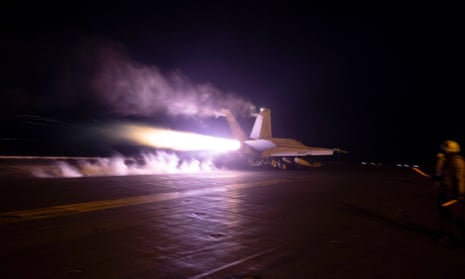This nighttime image captures a dramatic scene on an aircraft carrier where a white jet is poised for takeoff. The black sky and dark runway create a stark contrast against the intense white-hot flame blasting out of the jet’s exhaust, which lights up the surrounding area and leaves a luminous trail behind. Smoke billows from the jet's wheels as they speed along the runway, emphasizing its rapid acceleration. Off to the right, a flight deck officer is visible, partially illuminated by the jet’s glow. Dressed in a white hat, reflective vest or jacket, and black pants, he holds light sticks to direct the jet’s path. In the distant background, faint lights, possibly from the carrier or another source, shimmer subtly in the darkness, adding depth to the scene. Despite the low resolution, the image powerfully conveys the motion and intensity of the jet's takeoff.